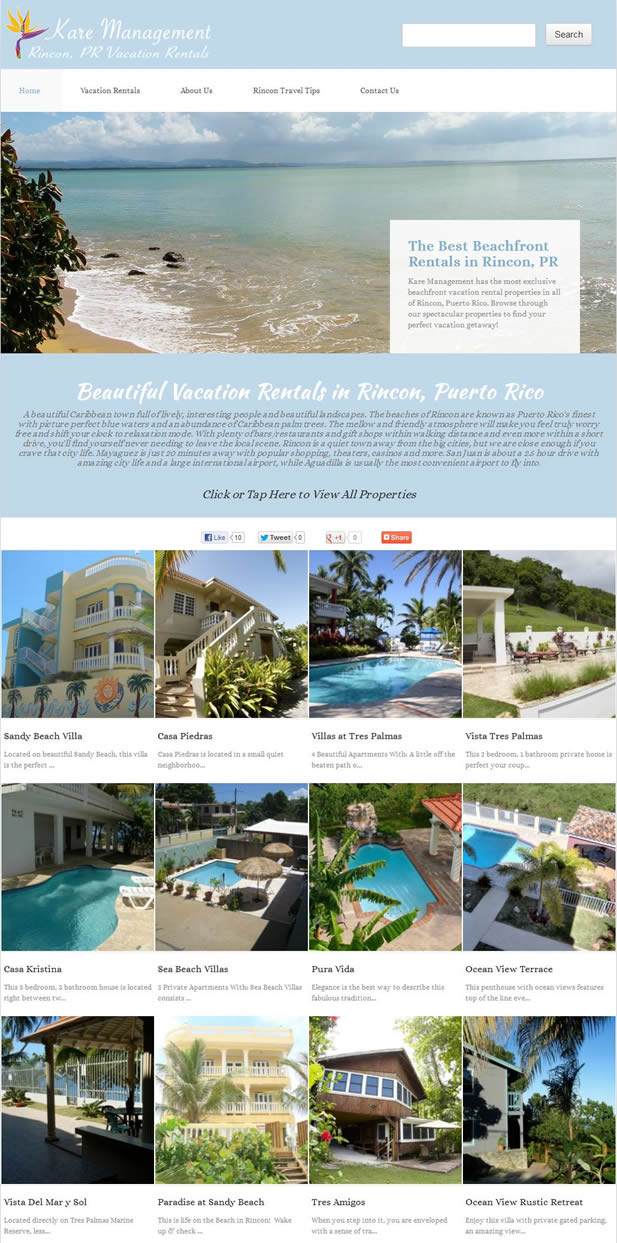In this image, we observe a detailed screenshot of a webpage titled "KARE Management," with "KARE" spelled in capital letters. The emblem to its left is designed in purple and yellow hues, resembling a flower. Below the title, there’s a picturesque beach photo featuring a vast blue lake with visible waves crashing against the rocks by the shoreline. On the left side of the image, there is a sandy shore accompanied by a green succulent plant.

The headline within the webpage reads: "The Best Beachfront Rentals in Rincón, PR," where "PR" stands for Puerto Rico. Below the headline, it confirms the destination with the text: "Beautiful Vacation Rentals in Rincón, Puerto Rico." A small, unreadable block of text follows before an actionable link that reads: "Click or tap here to view all properties."

The webpage displays a grid showcasing 12 properties in total, arranged in a format of four columns and three rows. Detailed descriptions of these properties include:

1. A yellow house with two-story porches, white stairs on the exterior, a wall adorned with palm tree murals, and a painting of a yellow and orange flower.
2. A property with a long angled stairway leading up to a two-story building that includes a garage or opening at the bottom and a door on one side.
3. A large pool beside a two-story house located on the far left with palm trees overhead and a clear blue sky.
4. A white structure that appears to be a covered area with a white wall, a green grassy lawn, and trees in the background.

In the second row:

5. A curved pool adjacent to a shaded, covered portion of a house.
6. Another pool with large beach umbrellas encircling it and bushes growing around two sides.
7. A large, uniquely shaped pool with semicircular curves at the top and bottom ends, adorned with palm trees.
8. A house with palm trees, a white fence, and a small rectangular pool.

In the third row:

9. A covered shaded area, lacking a pool but equipped with a bench-style table and a white fence.
10. A three-story yellow building with a palm tree matching its height, steps leading up to the house, and green shrubbery in front.
11. A two-story brown building with a large row of windows, featuring white frames and possibly sky-reflecting grayish-blue panes.
12. A gray house on the left set against a blue sky, some palm trees, and ground cover.